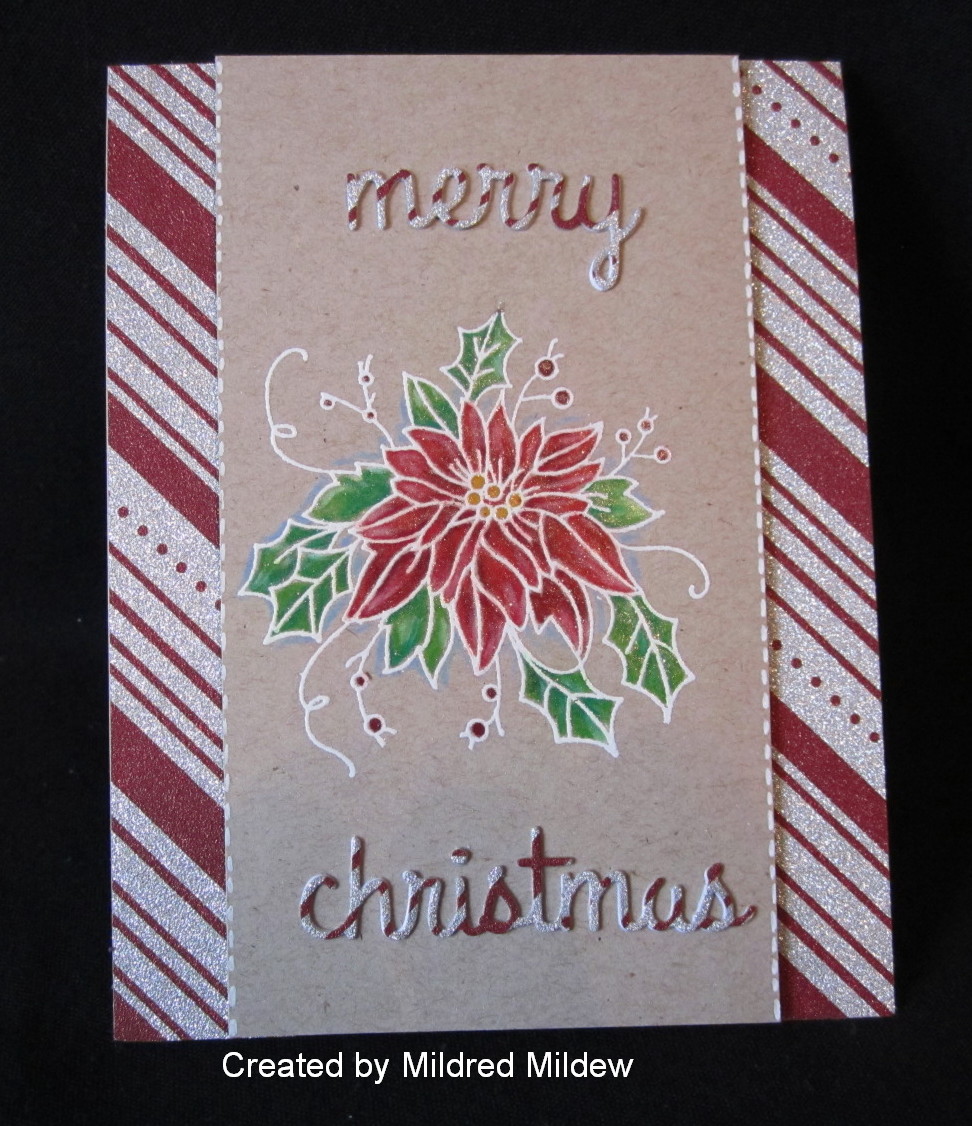The photograph captures a Christmas card resting on a black frame. The card's design features red and white candy cane stripes running vertically along both the left and right edges. The central section has a beige, natural paper look, giving it a rustic feel. Prominently displayed in the middle is a hand-drawn poinsettia, surrounded by green holly leaves and red holly berries. The poinsettia showcases vibrant red petals with a yellow center. Above and below the flower, the greeting "Merry Christmas" is written in cursive, with the lettering styled in red and white candy cane stripes, giving it a 3D effect. At the bottom of the card, in white font, is the text "Created by Mildred Mildew." The whole card lies flat against a black background, emphasizing its festive design.